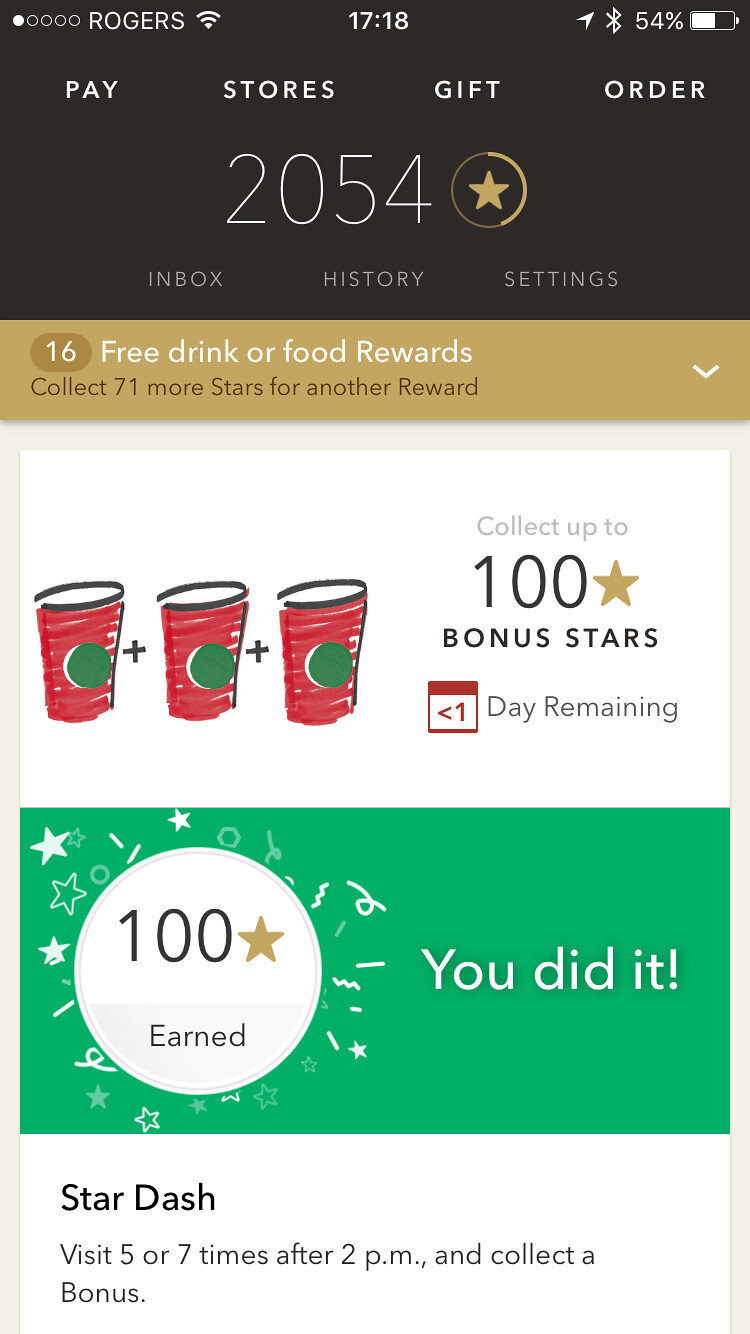The image is a screenshot of a mobile app, likely related to a rewards program, possibly for a coffee shop like Starbucks. At the top of the screen in a black bar, it displays 'Rogers' (presumably the carrier), the time '1718' (5:18 PM), and the phone's battery at '54%'. Just below, there are options labeled 'Pay', 'Stores', 'Gift', and 'Order'. The user's account shows '2054' points and indicates '16 free drink or food rewards'. To earn another reward, the user needs to collect '71 more stars'.

A central tan strip highlights the reward status and mentions, "collect up to 100 bonus stars, one day remaining," along with three red cups decorated with green dots. Below this section, against a green background, there's a congratulatory note: '100 stars earned', 'You did it!'. The bottom section, in white text, promotes the 'Stardash' challenge, encouraging visits "five or seven times after 2 PM" to collect a bonus. The main colors utilized in the app are white, red, green, tan, and dark brown.